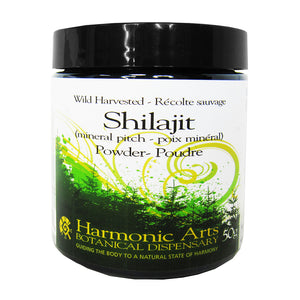The image features a small, round plastic container with a black lid, labeled in a white background with intricate green and yellow gradient designs. The top of the label displays the words "Wild Harvested, Recolite, Sauvage" in small black text, followed by "Shilajit" in larger black text, which stands for a mineral pitch and powder product. Beneath "Shilajit," there is additional text indicating it as "Mineral Pitch," accompanied by foreign language text likely reading "Poix Mineral." The label includes a blend of green and yellow hues, with a digitally created swirl transitioning from green at the bottom to yellow-green at the top, framing an image of green trees. The bottom part of the label reads "Harmonic Arts, Botanical Dispensary" in yellow text, adjacent to a yellow symbol resembling a capital G or a decorative swirl. Despite some smaller text being unclear, it appears to convey a message about restoring the body to a natural state or harmony. The overall composition suggests this product is marketed as a supplement, with the clean white background enhancing its presentation.